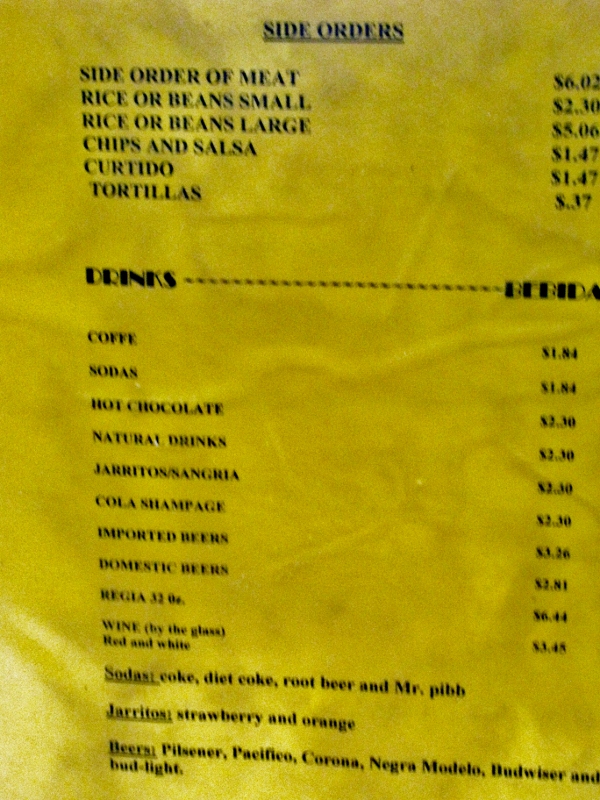This detailed image caption for the menu reads:

---

The menu is printed on yellow paper with black text. At the top, a heading reads "Side Orders," underlined by a bold black line for emphasis. Listed below this heading are the following side orders with their respective prices: meat ($6.02), small rice or beans ($2.30), large rice or beans ($5.06), chips and salsa ($1.47), curtido ($1.47), and tortillas ($0.37).

Following the side orders, the section titled "Drinks" features various beverage options: coffee ($1.84), hot chocolate ($2.30), natural drinks ($2.30), Doritos Sangria ($2.30), cola champagne ($2.30), imported beers ($3.26), domestic beers ($2.81), Regia 32-ounce beer ($6.44), and wine by the glass, available in both red and white varieties ($3.48). 

The selection of sodas includes Coke, Diet Coke, Root Beer, and Mr. Pibb. Additionally, the Doritos beverage options are available in strawberry and orange flavors. The beer selection comprises Pilsner, Pacifico, Corona, Negra Modelo, Budweiser, and Bud Light.